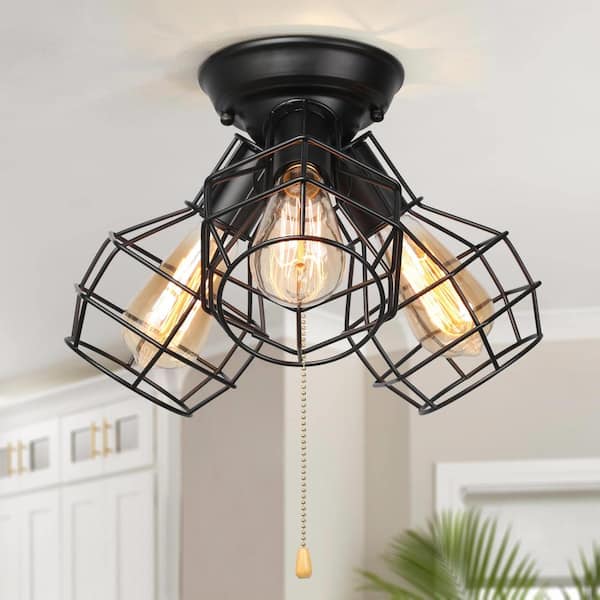This indoor photograph showcases a flush mount ceiling light fixture with a black metal base. The centerpiece of the fixture is a pole chain featuring a small brown knob at its bottom, used to turn the light on and off. The fixture hosts three Edison bulbs, each encased in a distinctive black wire cage with a grid-like structure reminiscent of bird cages. These light bulbs, cylindrical and tapered at the ends, emit a warm yellowish-gold glow. They are arranged in a triangular layout, spreading outward from the central base. The room itself has white ceilings and a creamy beige painted wall. To the left of the light fixture, there is a pair of white doors with windows above, while the right-hand corner features a window adjacent to a green plant.